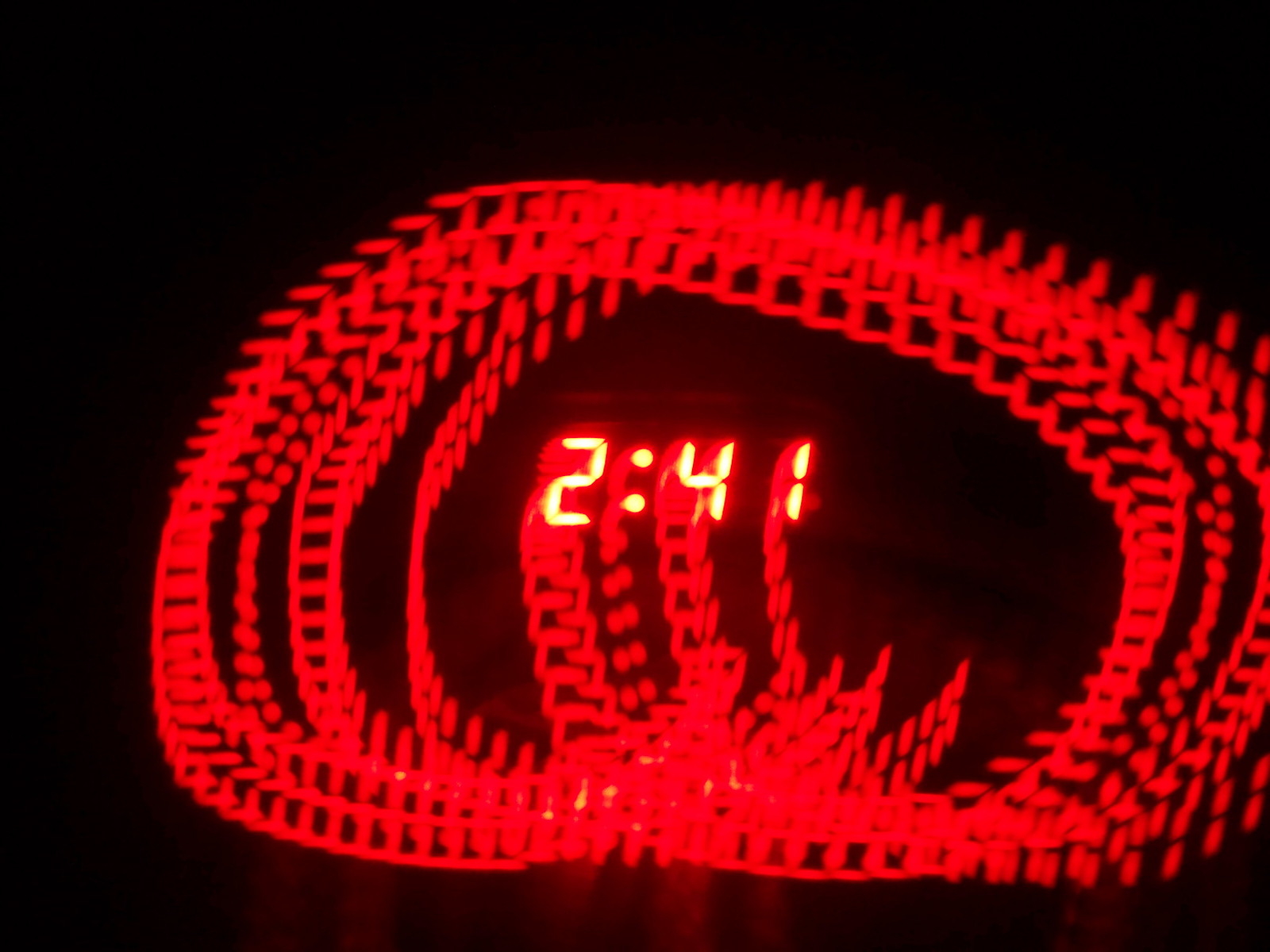The image is a heavily stylized color photograph captured in a blackened room where an LED digital clock reads "2:41" in a yellowish-red hue. The photograph appears to have been either taken with a long-exposure technique or digitally manipulated afterward. From the centrally positioned LED readout, numerous lines that make up the digits cascade downwards and then spiral in an oval pattern, seemingly tracing the path of the clock's movement. These lines are incrementally spaced, creating segmented arcs that encircle the initial display. The movement of the clock, possibly achieved by purposefully shaking and rotating the camera, has left a vivid red streak that loops around multiple times, forming a complex, swirling pattern. The background remains a deep, impenetrable black, with slight bleeding highlights emanating from the spiral of dotted lines, fading gradually into the darkness. There are no other visible elements, text, or artist marks in the image, emphasizing the artistic and experimental nature of this striking visual effect.